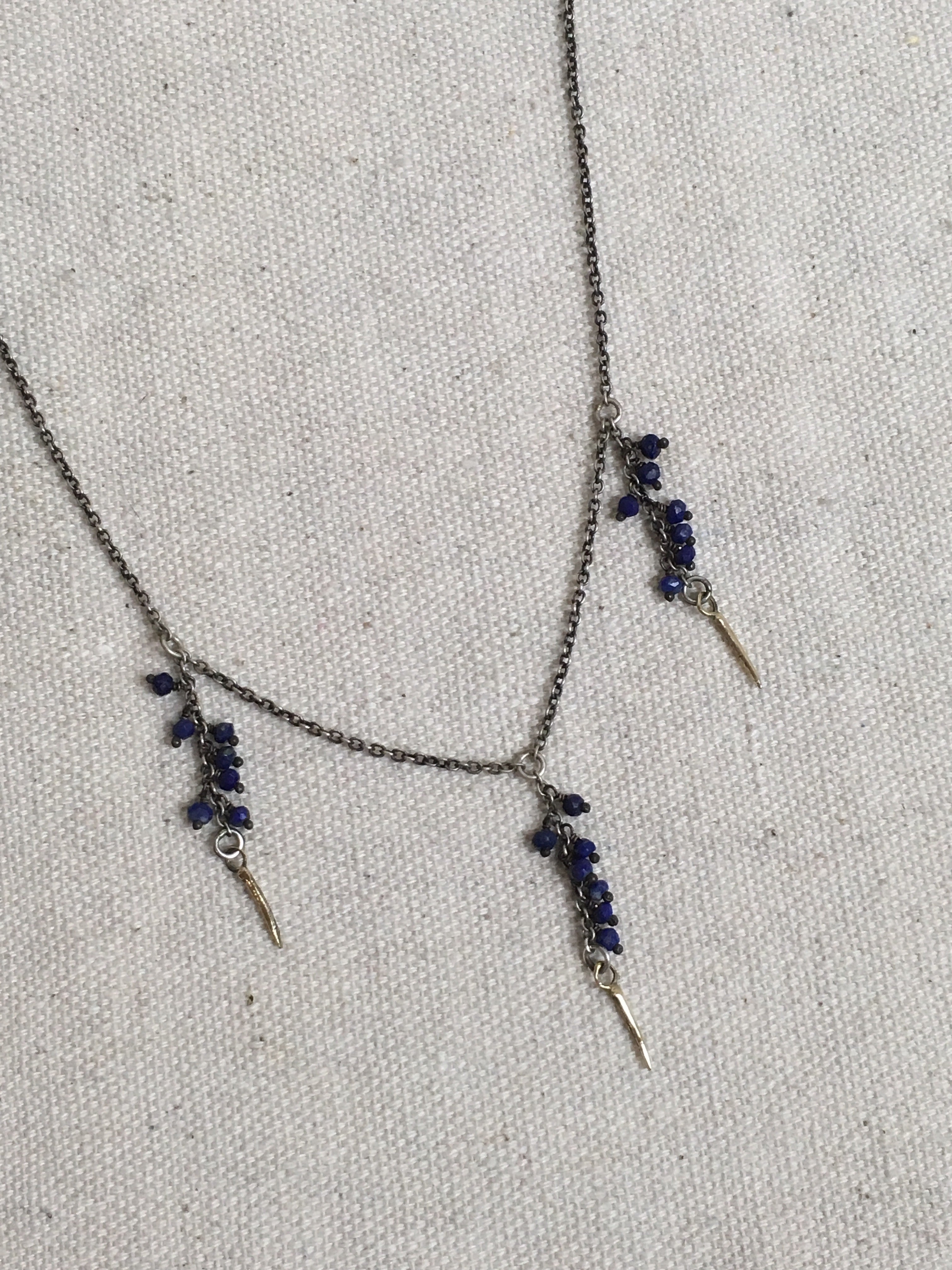This vertically aligned rectangular image features a chain necklace laid atop a white fabric with tiny black specks, creating a vented or dotted pattern. The chain, which navigates the frame from the top center and left middle, is a blackish-silver color, though hints of gold could also be perceived. Three distinct pendants dangle from the necklace: one on the left, one in the middle, and one on the right. Each pendant consists of small black beads or flower-like objects linked together, culminating in a silver pointed tip or shaft at the bottom. The left pendant appears to have seven of these black elements, the middle pendant features six, and the right pendant, seven again, all varying slightly in size. The detailed arrangement gives the necklace an ornate and intricate appearance, suitable for a jewelry advertisement.